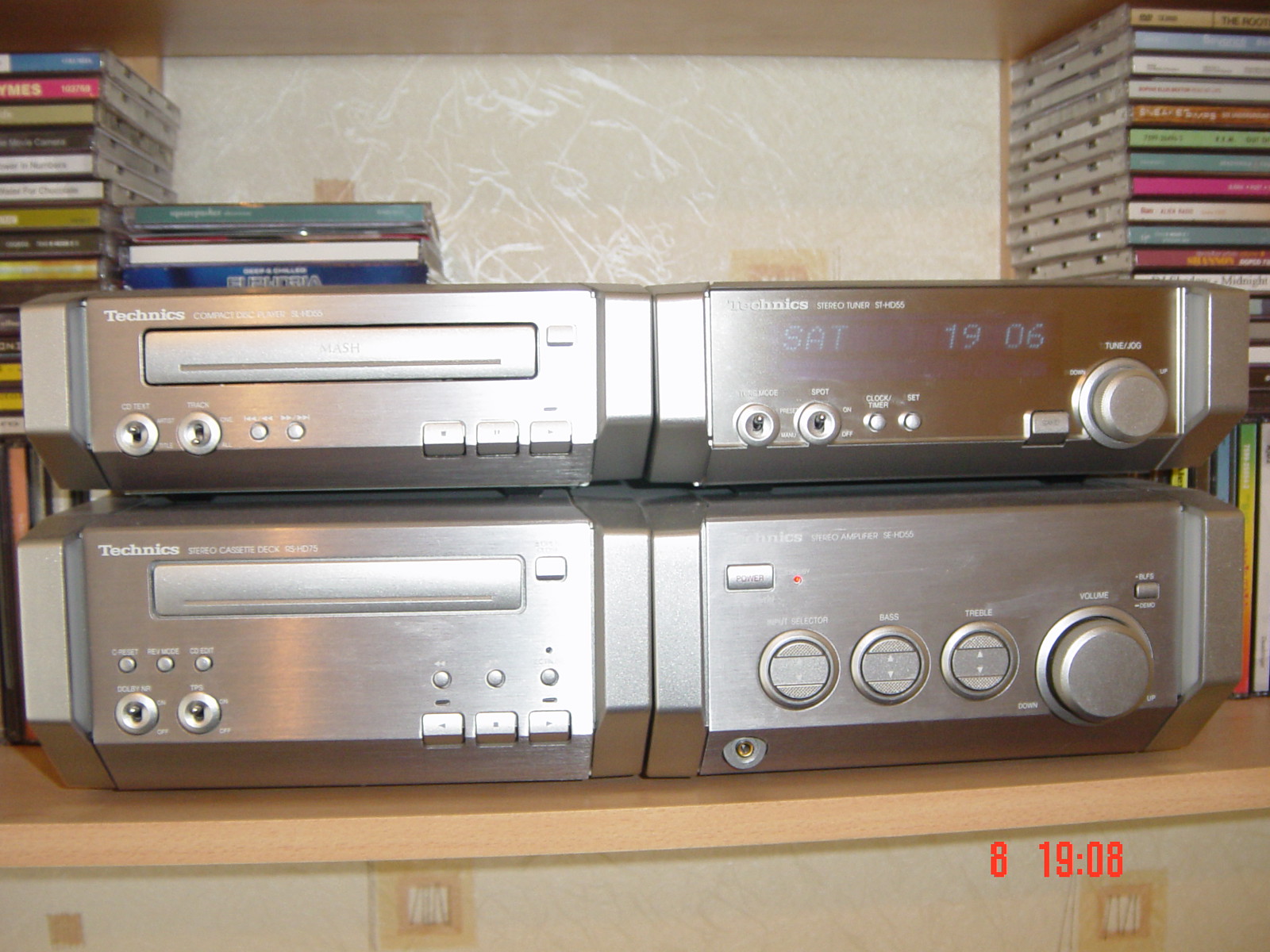This photograph captures a vintage Technics stereo system from the 1990s, prominently featuring two stacked units, both in a silver chrome color. The upper unit displays a digital readout of "SAT19..06" and both units have the brand's logo visible on the middle right and far left areas. The bottom unit is noticeably thicker and includes a stereo cassette deck, which indicates it can play cassettes, in addition to potentially handling radio functions. Both units include a CD player on the left side and various tuning dials on the right. These stereo components occupy the majority of the image, horizontally stretching across it.

The system rests on a light beige wooden shelf, which is nailed to a textured ivory wall adorned with streaks and lines. The background is filled with vertically stacked CDs, some featuring Asian script on their spines. Three CD stacks reach almost up to the bottom of the next shelf, while another stands slightly shorter. Beneath the devices, a light yellow-tan counter or table with a faint wood grain is visible. This entire setup suggests a nostalgic music lover’s corner, showcasing a blend of past media technologies.